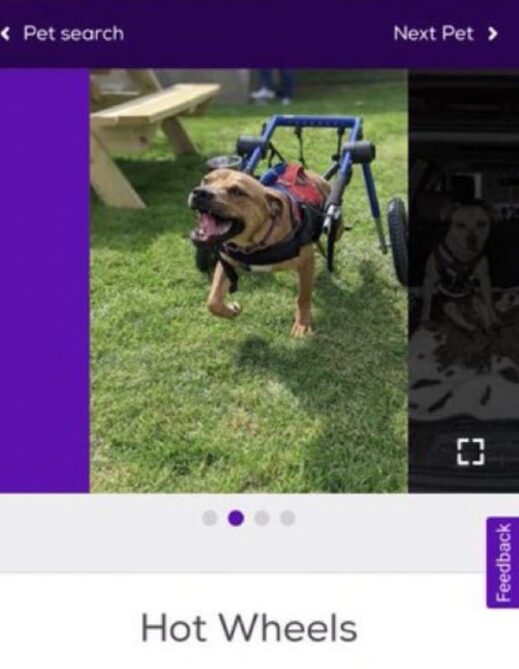The image features a dark purple header at the top, with a left-pointing arrow labeled "Pet Search" on the left side and a right-pointing arrow labeled "Next Pet" on the right side. Below the header, on the left-hand side, is a long, lighter purple rectangle. Adjacent to this rectangle is an image of a dog harnessed to a wheeled contraption, suggesting the dog may be using it to assist with mobility. Further below, there is a faint gray rectangle containing another dog, though the details are obscured and it is difficult to identify what else is depicted within this section.

Additionally, the image includes a semi-square shape with small gaps at the center of each side, housing a series of smaller shapes. These include a central gray circle, flanked by alternating gray and purple circles. On the right-hand side, there is a gray rectangle labeled "Feedback." At the very bottom of the image, the text "Hot Wheels" is displayed, possibly hinting at the wheeled contraption associated with the first dog. The overall layout appears to be part of an interface for browsing or searching through pet profiles, with navigation and feedback options integrated into the design.